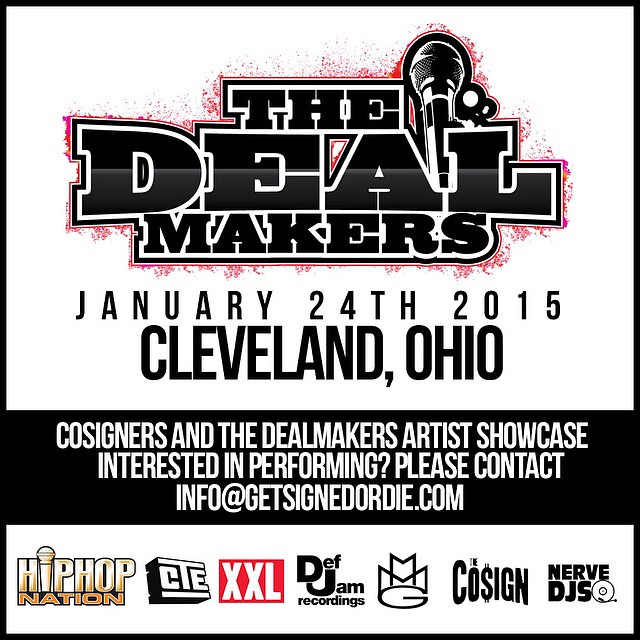The image is a square advertisement poster with a predominantly white background and a black border. At the top, it displays the bold, stylized text "The Dealmakers" in unique black graphic art font, incorporating a black microphone into the design. Below this header, it provides details about the event: "January 24, 2015, Cleveland, Ohio," all in black text. Further down, a black strip with white letters reads, "Co-signers in the Dealmakers Artist Showcase. Interested in performing? Please contact info@GetSignedOrDie.com." At the bottom of the poster, various logos of prominent sponsors and recording companies such as Hip Hop Nation, CTE, XXL, Def Jam Recordings, MMG, The Co-sign, and Nerve DJs are displayed, featuring a mix of colors and designs.